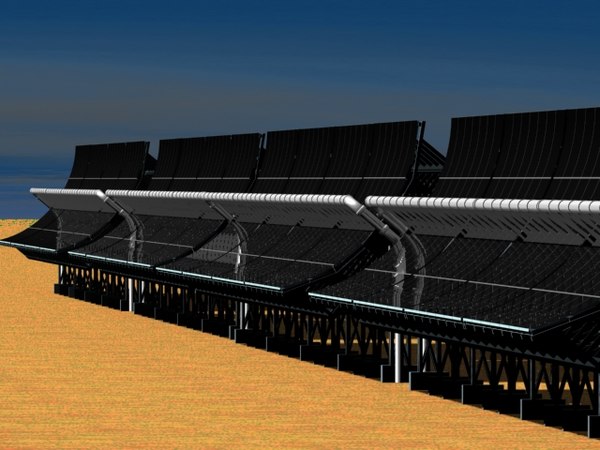The image depicts a detailed, computer-generated rendering of four large, black solar panels situated in a desert-like plain with yellowish sand. The sky above is dark blue with light, dark-gray clouds blending into it. The solar panels, which dominate the majority of the image, are distinctive with their slight curve and bend, transitioning from a curved shape at the bottom to an upright stance. The panels are oriented from right to left, appearing larger on the right and smaller on the left. Notably, silver channels run through the center of each panel, potentially functioning as light reflectors to enhance their efficiency. This intricate setup against the stark, expansive landscape and the vibrant sky further emphasizes the advanced and futuristic design of the solar energy installation.